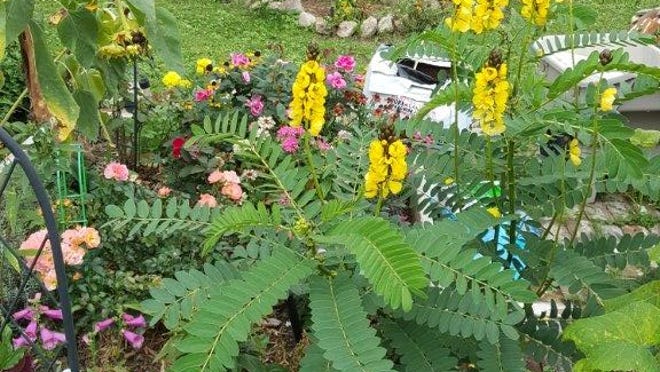This vibrant and detailed garden scene is bustling with a diverse array of plants and flowers. Dominating the foreground is a lush green fern, its fronds elegantly splayed out. Just behind the fern, a tall yellow-flowered plant reaches upwards, reminiscent of snapdragons. Intermingling with these are small carnations in pink, red, and yellow hues, adding splashes of color. On the lower left-hand side, a stunning purple hollyhock makes an appearance.

Green grass extends beyond this rich tapestry of flora, framing a section with mulch encircled by a neat ring of gray stones in the background. To the right, the corner of the image captures an iron mesh structure and a charming brick walkway, hinting at the garden's well-maintained pathways. Heart-shaped green leaves with brown stems and blue flowers peek through the greenery, contributing to the garden's layered and textured appearance. Scattered throughout are various shades of green and brown, alongside vivid floral colors, creating a cheerful and inviting setting that exudes the charm and tranquility of a thoughtfully cultivated backyard sanctuary.